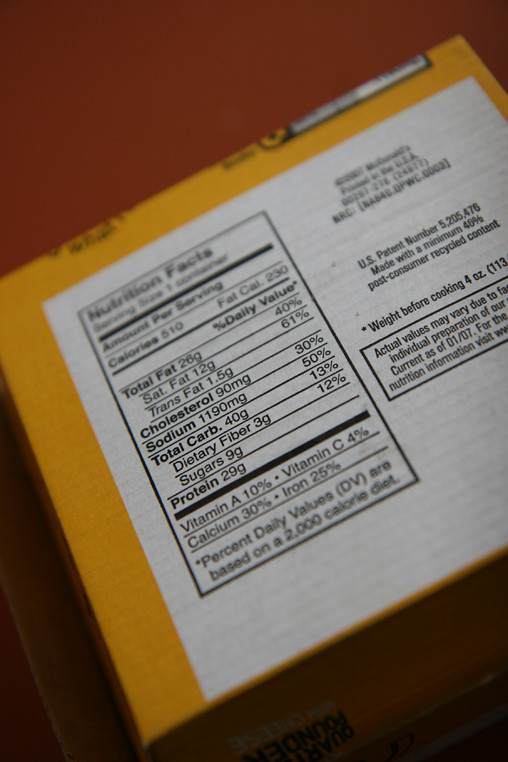The image displays a McDonald's burger box with a distinctive square shape. The box has a yellow rim and a white inner square, emblazoned with black lettering. On the left side of the box, there is a nutrition facts label, while the right side contains consumer information confirming its origin from McDonald's. The photo is taken at a slightly slanted angle, with a red table in the background adding a splash of color.

Examining the details, the box states it is made with a minimum of 46% post-consumer recycled content. It bears a USA label and a patent number, providing the weight before cooking as 4 oz, although actual values may vary due to individual preparation. The current information mark is 01-7, and part of the nutrition information is slightly cut out of the photo.

The nutrition facts label specifies that the serving size is one container, with a total caloric content of 510 calories. Of these, 230 calories come from fat. The detailed breakdown is as follows: Total fat is 26g, saturated fat is 12g, trans fat is 15g, cholesterol is 90mg, sodium is 190mg, total carbohydrates are 40g (including 3g of dietary fiber and 9g of sugars), and protein content is 29g. Additionally, the nutritional percentages include 10% of the daily value for vitamin A, 4% for vitamin C, 30% for calcium, and 25% for iron. The box highlights the substantial nutritional content and reflects a typical fast-food item, characterized by its high-calorie and high-fat content.